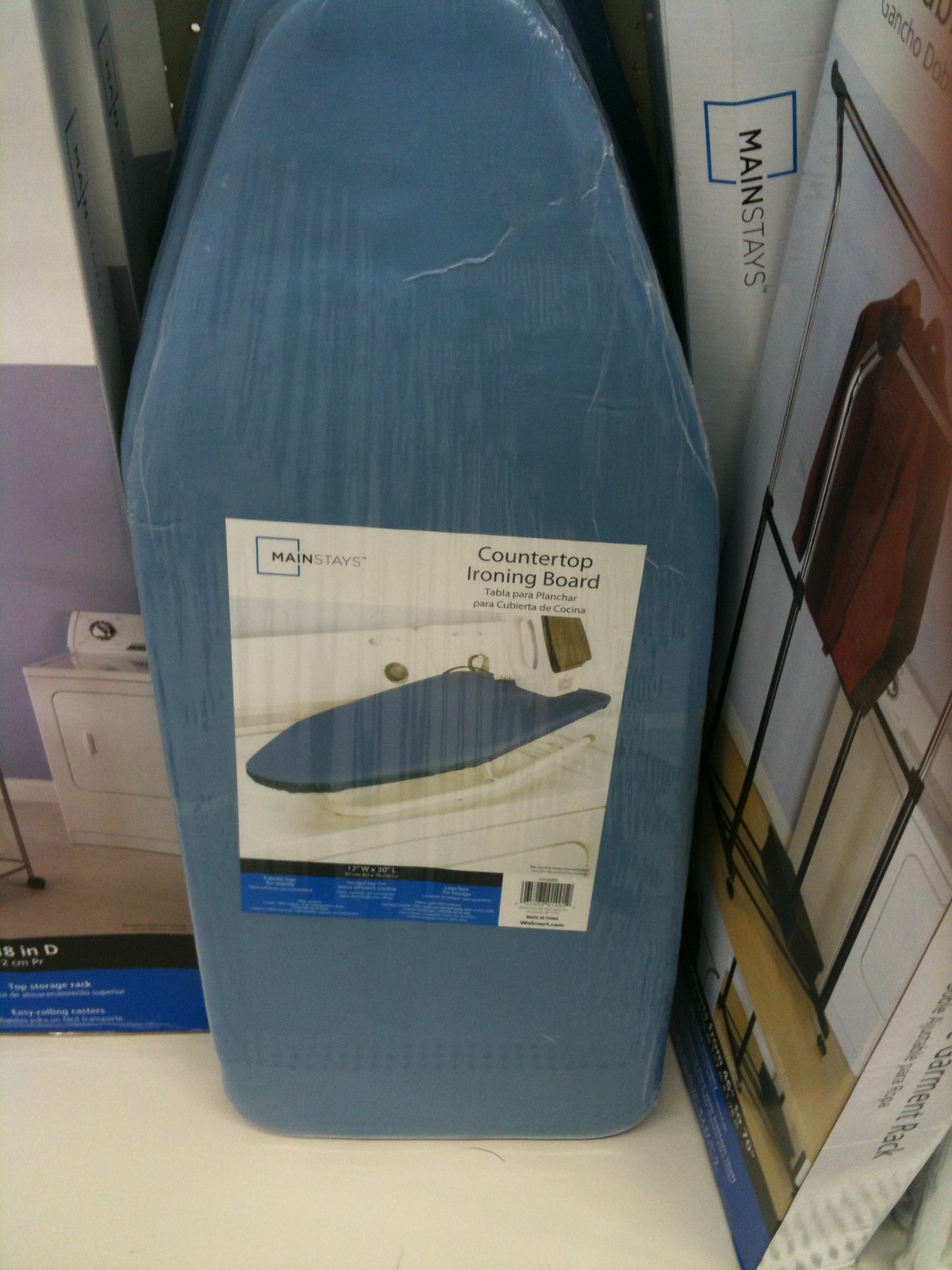This color photograph, taken in a homewares store, likely Walmart, is in a portrait orientation and focuses primarily on a shrink-wrapped countertop ironing board cover. The cover is turquoise blue and designed by the brand "Mainstays." The ironing board is slightly cut off at the top, but a piece of paper label underneath the shrink-wrap is visible, reflecting light. The top right of the label reads "countertop ironing board" in black text, and it includes an illustrated example of the cover in use. The top left features the "Mainstays" logo, and the bottom right has a barcode. The ironing board has short, white extendable legs. To the left, out of focus, are several identical long boxes with geometric shapes and patterns, containing other homeware items, possibly a clothing rack, adding to the impression that this scene is set in a store selling practical home goods.